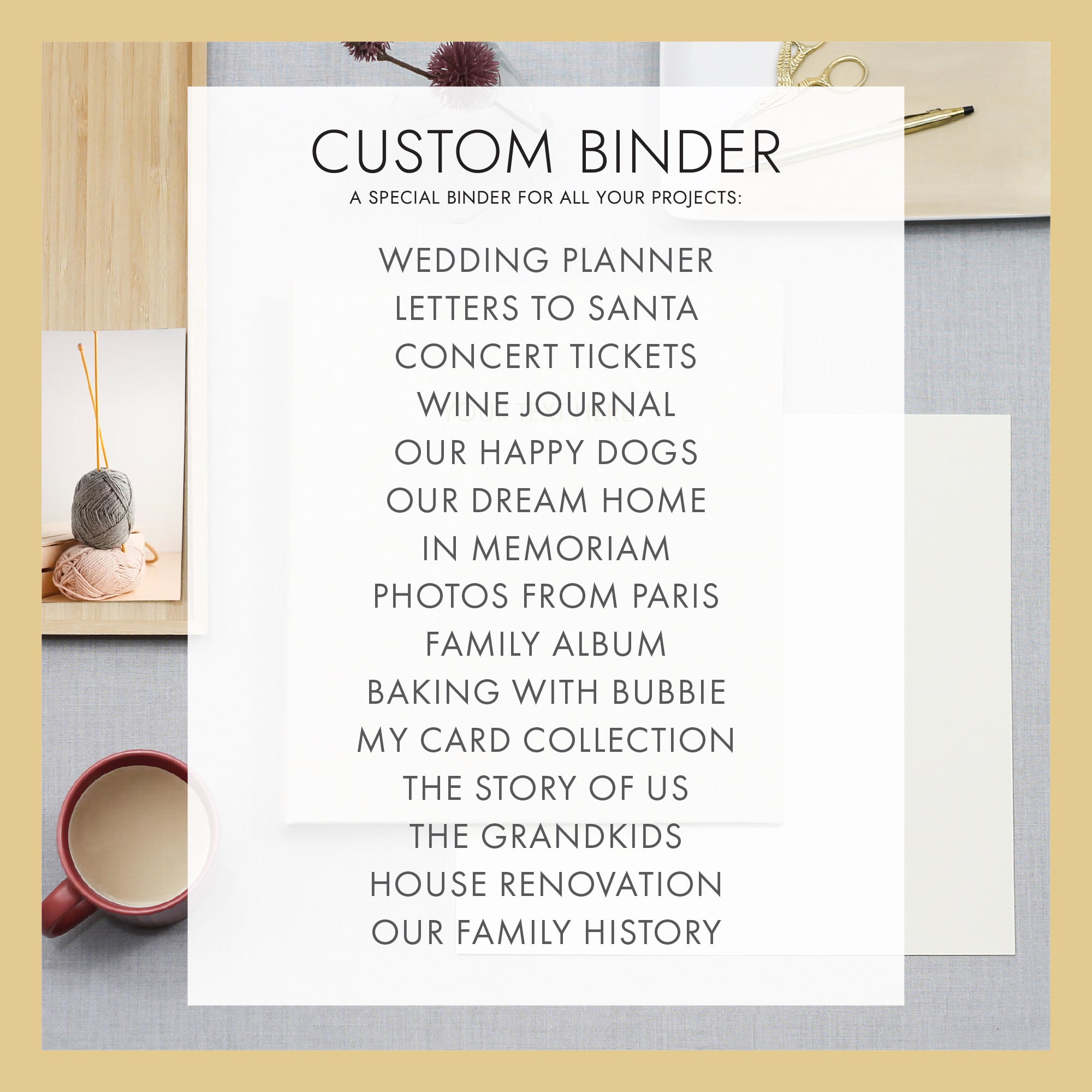The image is an advertisement for a custom binder, designed to organize various personal projects. The background is a rich collage of photographs featuring a mix of crafting and lifestyle elements. Central to the composition is a semi-transparent white rectangle with black text. At the top, bold sans serif capital letters state, "CUSTOM BINDER," followed by the smaller text, "a special binder for all your projects." Below this, a series of potential uses for the binder are listed, including "Wedding Planner, Letters to Santa, Concert Tickets, Wine Journal, Our Happy Dogs, Our Dream Home, In Memoriam, Photos in Paris, Family Album, Baking with Bubby, My Card Collection, The Story of Us, The Grandkids, House Renovation, Our Family History."

The collage around this text includes a coffee mug on a gray surface next to a white sheet of paper in the lower left corner. Adjacent to it is a photograph featuring two balls of yarn—one pink and one gray—with knitting needles inserted into the gray yarn. At the top of the image, a pair of gold scissors lies next to a golden pen, and a purple flower adds a touch of natural elegance. This visually rich background beautifully complements the practical and versatile message of the custom binder, inviting viewers to organize their cherished memories and projects in a stylish manner.